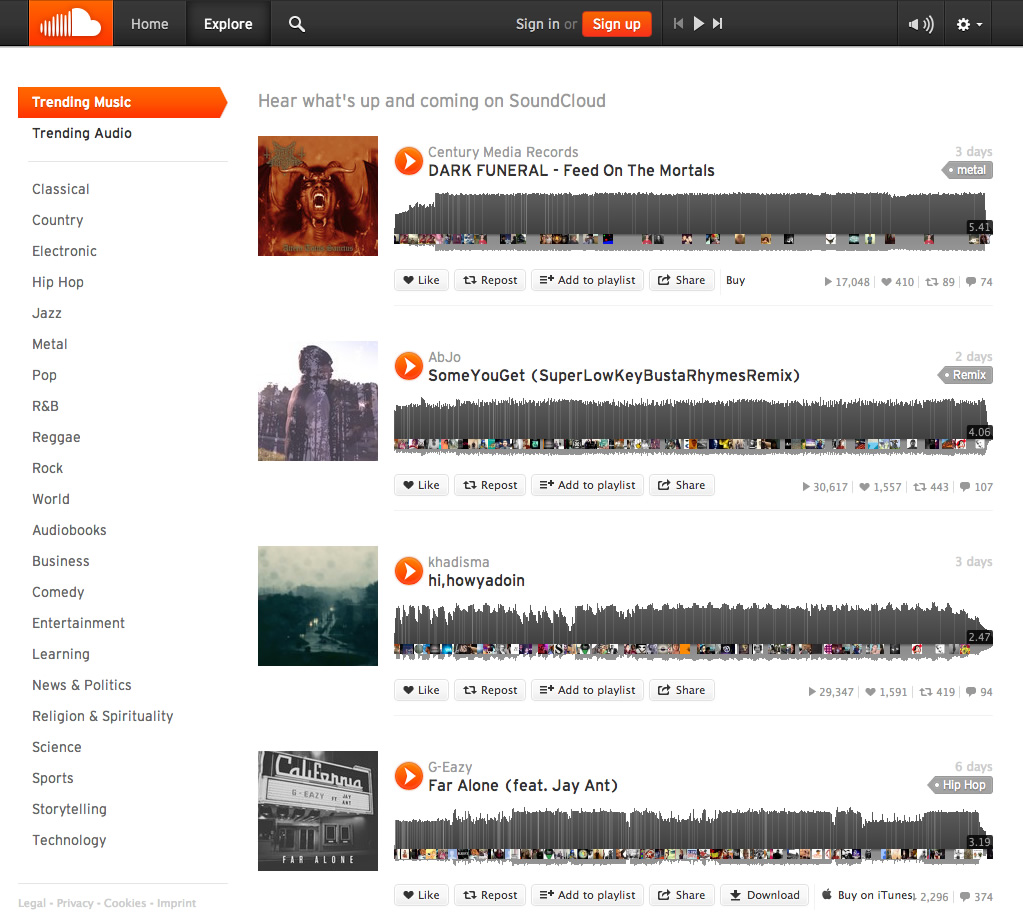The image features a website interface, prominently displaying the recognizable orange icon of SoundCloud in the top left corner, indicating that this is indeed the SoundCloud platform. A black bar spans horizontally across the top of the page, offering navigation options such as "Home," "Explore," a search bar, and buttons to "Sign In" or "Sign Up."

At the top of the page, user interface controls include a play button, a fast forward button, a sound button, and a settings button. On the left side of the page is an orange banner labeled "Trinity Music," with a clickable section beneath it titled "Trinity Audio."

Running down the left sidebar is a comprehensive list of genres written in gray, enabling users to explore a variety of auditory content ranging from Classical and Country to Electronic, Hip Hop, Jazz, Metal, Pop, R&B, Reggae, Rock, World, Audiobooks, Business, Comedy, Entertainment, Learning, News and Politics, Religion and Spirituality, Science, Sports, Storytelling, and Technology.

Highlighted on the main section of the interface are upcoming releases and featured tracks on SoundCloud. The featured content includes "Dark Funeral" by Century Media Records, a metal genre track titled "Feet on the Mortals," a super low key remix by Busta Rhymes, "Hi, How You Doin'" by Khadizma, and "Far Alone" by G-Eazy, which belongs to the hip hop genre. Users have a wide array of music and audio content to choose from on the platform.